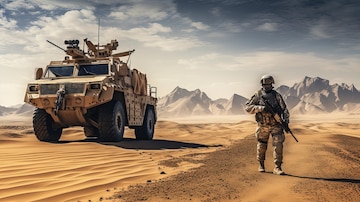The image is a small rectangular photo print of a desert scene. In the foreground, light brown sand covers the ground, with distinctive rocky patches on the right and wave-like ridges on the left. A soldier dressed in light brown camouflage, wearing a helmet and goggles, and holding a black rifle, is positioned towards the right side of the image. He appears to be walking towards the viewer. To the left of the soldier, there's a light tan military vehicle resembling a Humvee, equipped with large black wheels and mounted guns. The background showcases a gray and black mountain range under a predominantly dark gray sky with blue patches and clouds, which are more concentrated on the left side of the image.